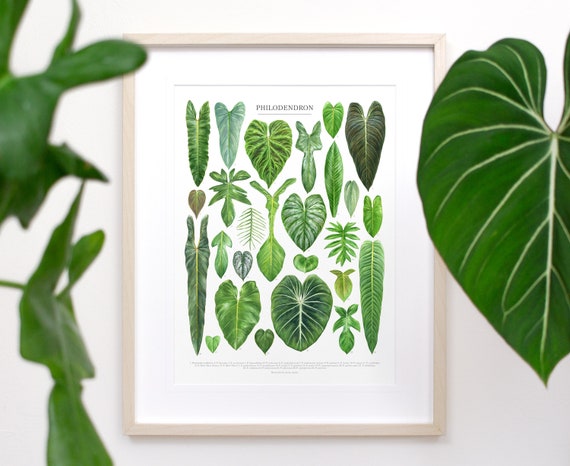The image depicts a well-lit indoor setting with a picture of a botanical chart in a wooden frame hanging on a white wall. The chart, labeled "PHILODENDRON" at the top in capitalized black letters, features a couple dozen different types of leaves arranged in a visually appealing manner. These leaves vary in shape, size, and shades of green—ranging from dark to light—along with some brown, tan, and off-white hues. The main focus of the image is this framed picture, which is primarily white in its border and background, providing a clear and detailed view of the diverse leaf specimens. Additionally, in the foreground, there are some leaf details captured in a close-up, adding an interesting layer to the composition. The setting is bright, filled with natural sunlight, enhancing the clarity and color accuracy of the photograph.